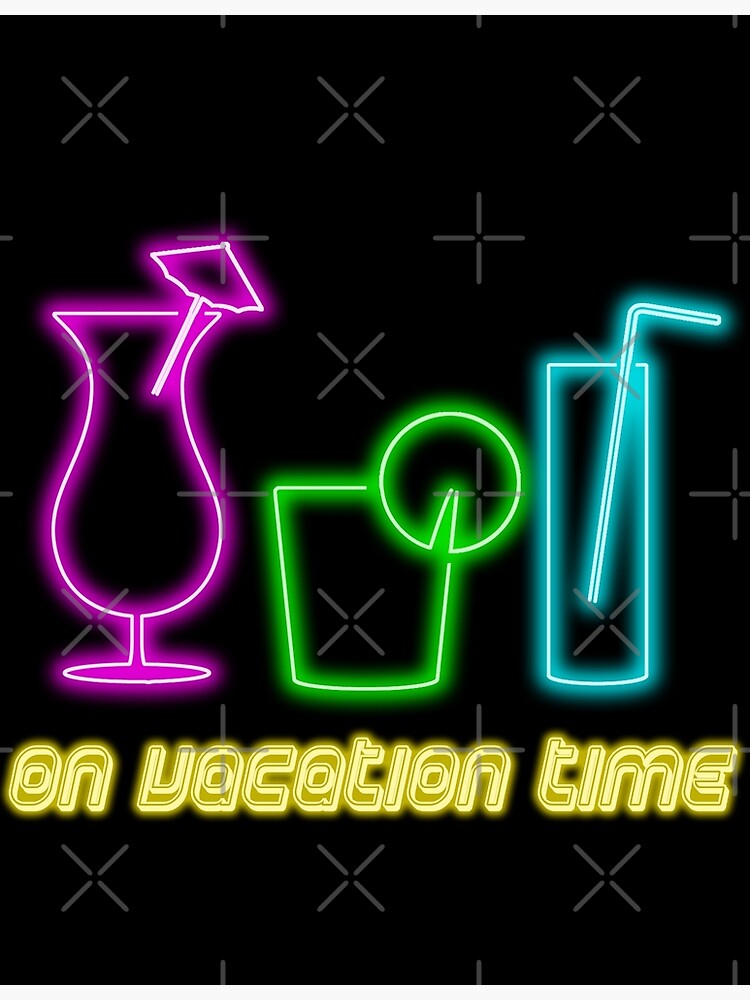The image features a neon sign set against a jet-black, opaque background adorned with a light gray watermark of X's and plus signs, likely to prevent unauthorized use. Three vividly neon-lit tropical beverages dominate the rectangular, horizontal composition. On the left, a vase-like neon purple glass is garnished with a small umbrella. In the center, a shorter neon green glass, possibly a shot glass, is embellished with a lemon or lime wedge. To the right, a tall, thin, neon blue glass with a straw completes the trio. Beneath these glasses, glowing in yellow and white neon lettering, is the phrase "On Vacation Time."